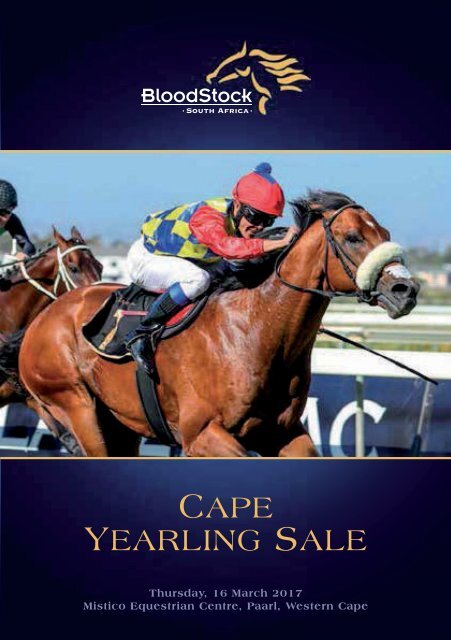The image depicts a dynamic scene of a jockey racing on a horse. The jockey, dressed in a distinctive outfit, wears a red cap with a blue top and a blue pom-pom, a red-sleeved shirt, and a blue and yellow diamond-patterned vest. He is also adorned in white pants and black boots. The jockey, small in stature, is leaning down close to his horse, adopting a racing posture. The horse, a striking brown with reddish tones, is captured mid-stride, running fast with the racetrack and another horse trailing in the background. Above, the text reads "Bloodstock South Africa" with a horse head logo. Below, additional text states "Cape Yearling Sale" followed by "Thursday, 16th March, 2017, Mystico Equestrian Center, Parral, Western Cape." The top and bottom text is set against a dark navy blue background. The image, centered on the jockey and horse, appears to be an advertisement or flyer promoting the event.